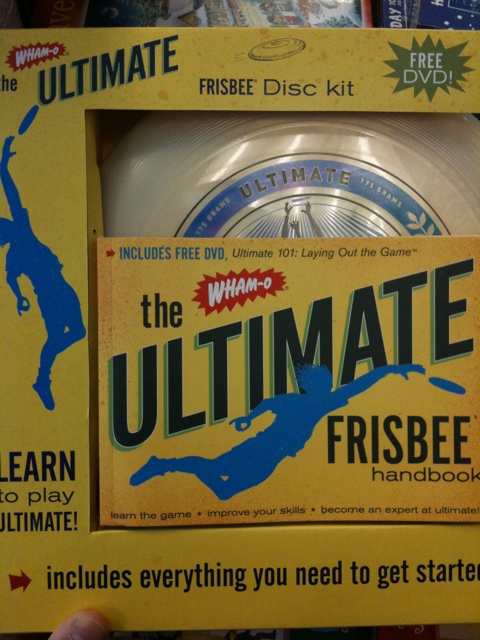This image showcases a detailed photograph of a yellow Ultimate Frisbee Disc Kit package, likely taken indoors, possibly within a store. Prominently displayed, the packaging highlights a white and blue Frisbee, prominently bearing the word "Ultimate". Above the disc, the package advertises a "Free DVD," detailing an introductory guide titled "Ultimate 101: Laying Out the Game." The Wham-O logo, marked in red and white spiky text, is clearly visible. Complementing the text are graphics of individuals actively engaged in playing Ultimate Frisbee—one diving and another jumping to catch a disc. The package also features phrases encouraging skill improvement and mastery of the game, such as "Learn the game, improve your skills, become an expert at Ultimate Frisbee." At the bottom, bold lettering ensures that the package includes all necessary components to get started. The left side of the image depicts a thumb holding up the box, adding a human element to the scene.